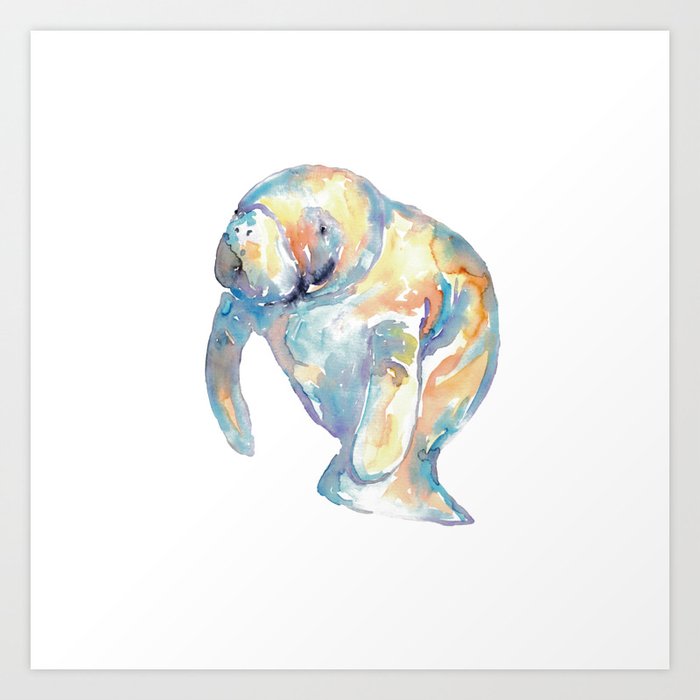This image displays a watercolor painting of an animal situated within a gray frame against a white background. The creature, which appears to be a manatee, stands upright, almost as if balanced on its tail, turned slightly to the left with its paddles or arms hanging at its sides. The painting employs an engaging mix of colors, blending turquoise, purples, blues, oranges, yellows, and even hints of pink in an ombre or tie-dye effect that gives a dynamic impression of light and shadow, perhaps reflecting sunlight. The manatee's expression seems somewhat melancholic, with distinct, small black eyes and subtle black markings around its mouth. The overall pastel color palette creates a soft and inviting visual experience. There is no text or signature from the artist visible within the artwork.